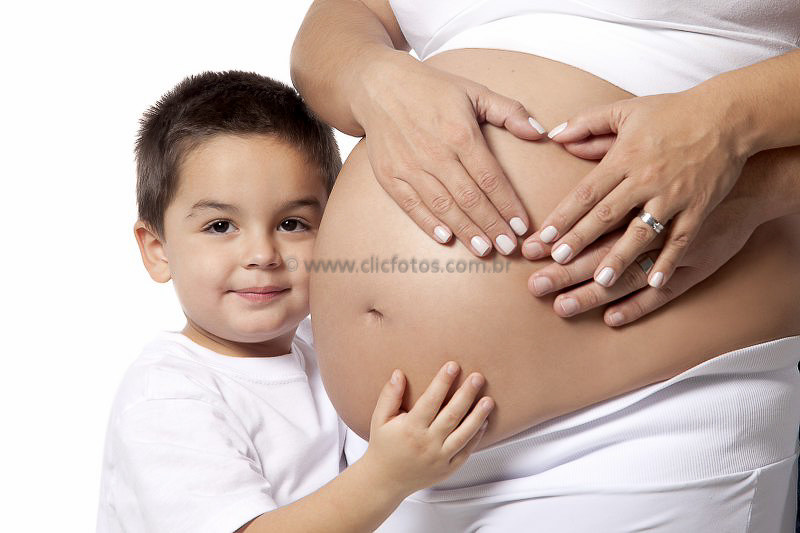In this detailed and touching photograph, a young boy with short, spiky brown hair and large brown eyes stands on the left side, tenderly touching his mother's large, bare pregnant belly. He is wearing a white crew neck t-shirt and looks directly at the camera with a closed-mouth smile. His mother's face is not visible, as the focus is on her exposed belly and the intimate moment shared with her family. Her attire includes a white shirt rolled up over her belly and white pants. Three hands, including the boy's, rest gently on her belly; two of them, likely the father's, are adorned with wedding bands and come from the right side of the image. The mother's hands, with white nail polish, lovingly cradle her stomach. The background is a solid white color, emphasizing the subjects, with a watermark reading "www.clickphotos.com.pr" positioned in the middle of the image.